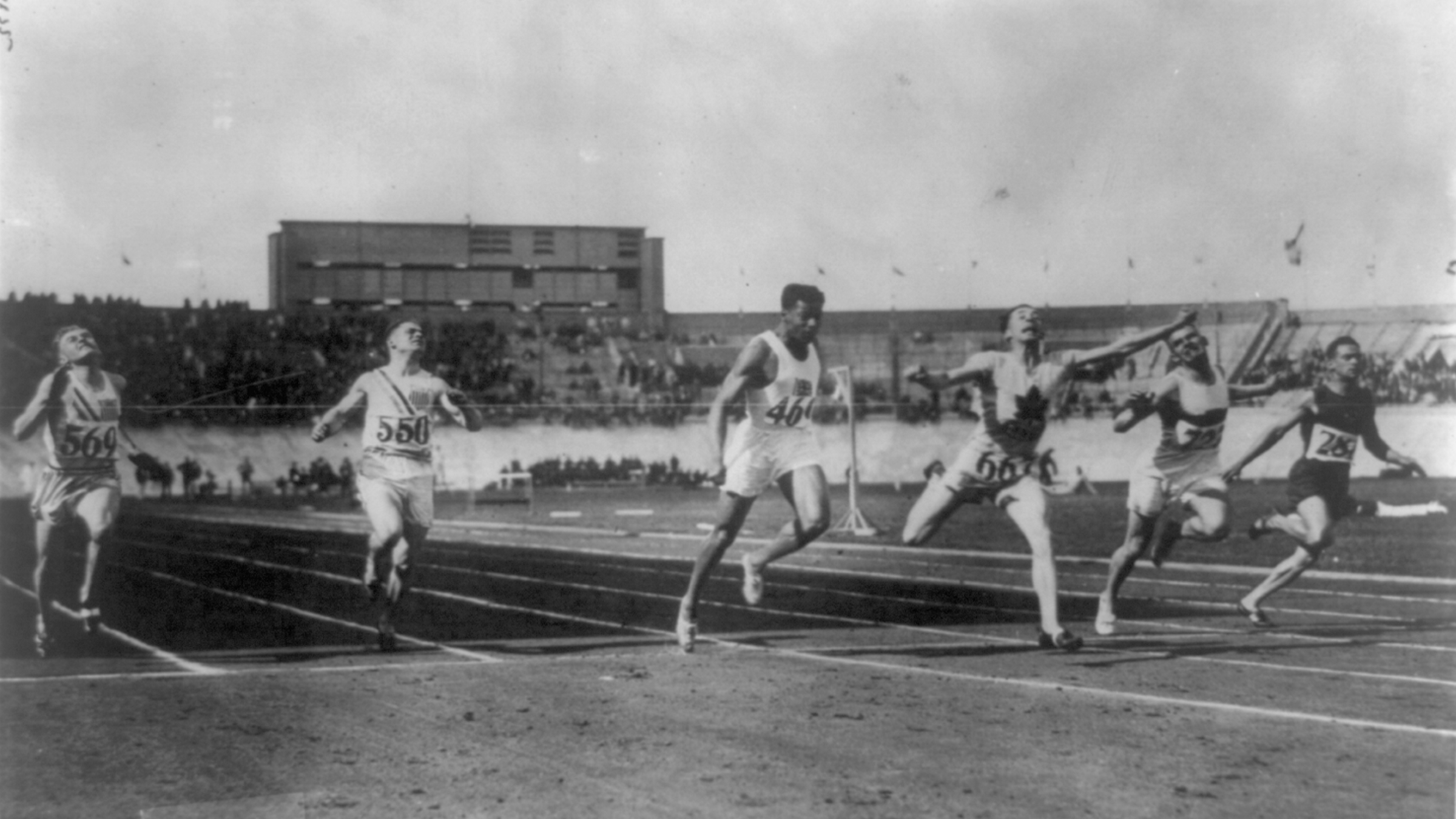This black and white, outdoor photograph captures a competitive foot race among six men on a racetrack with clearly marked lanes. Starting from the left, the runner in lane one is a white man wearing a bib numbered 569, his head tilted upward. Next to him in lane two, another white man, also looking up, sports a bib numbered 550. Lane three features a black runner, head down and wearing a partially legible bib starting with 46. The runner in lane four, a white man, has a bib numbered 66, possibly followed by another digit, and his arm is raised as he looks up. In lane five, another white man runs with an illegible number on his bib, his head also angled upward. Finally, the runner in lane six, wearing a black jersey and numbered 289, looks upward while dashing forward. The blurred background shows a cloudy sky and a stadium filled with spectators, enhancing the intense atmosphere of the race.